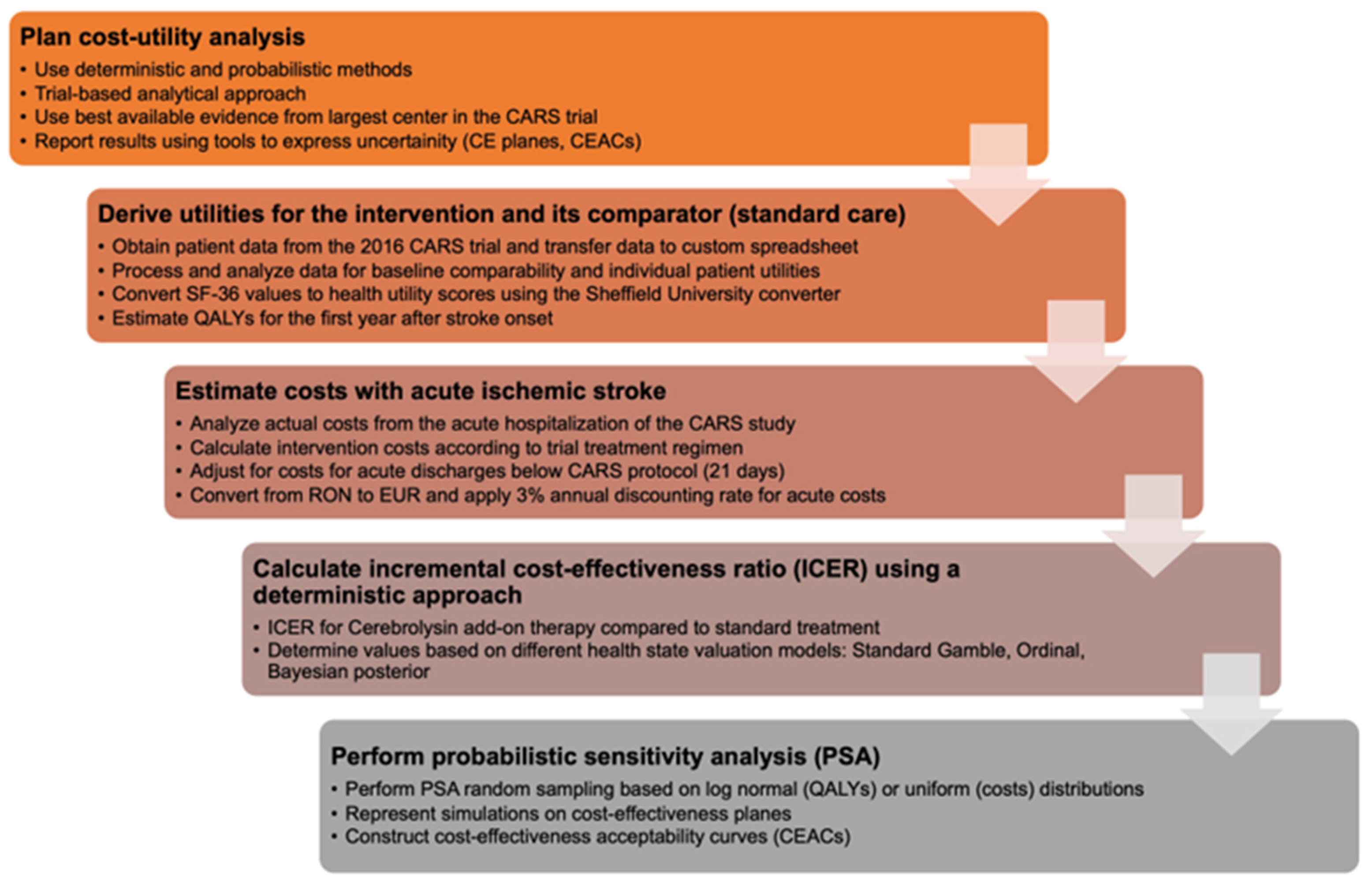The image is a detailed infographic structured as a vertical sequence of connected rectangles, each transitioning in color from bright orange at the top, through varying shades of orange and purple, down to a muted gray at the bottom. White arrows in each rectangle direct the viewer to the subsequent step. The first rectangle, titled "Plan Cost Utility Analysis," outlines the use of deterministic and probabilistic methods with trial-based analytical approaches, employing the best available evidence from the largest center in the CARS trial, and reporting results using tools like CE planes and CEACs to express uncertainty. The second rectangle, labeled "Derive Utilities for the Intervention and its Comparator Standard Care," involving obtaining patient data from the 2016 CARS trial, processing and analyzing this data for baseline comparability, and converting SF-36 values to health utility scores using the Sheffield University converter to estimate QALYs for the first year post-stroke. The third rectangle, "Estimate Costs with Acute Ischemic Stroke," describes analyzing actual costs from the CARS study, calculating intervention costs according to the trial treatment regimen, adjusting for early acute discharges, converting costs from RON to EUR, and applying a 3% annual discounting rate. The fourth rectangle, titled "Calculate Incremental Cost-Effectiveness Ratio (ICER) Using a Deterministic Approach," details calculating ICER for cerebral ozone add-on therapy compared to standard treatment using different health state valuation models like standard gamble, ordinal, and Bayesian posterior. The final rectangle, "Perform Probabilistic Sensitivity Analysis (PSA)," entails performing PSA with random sampling based on log-normal QALYs or uniform cost distributions, representing simulations on cost-effectiveness planes, and constructing cost-effectiveness acceptability curves (CEACs).